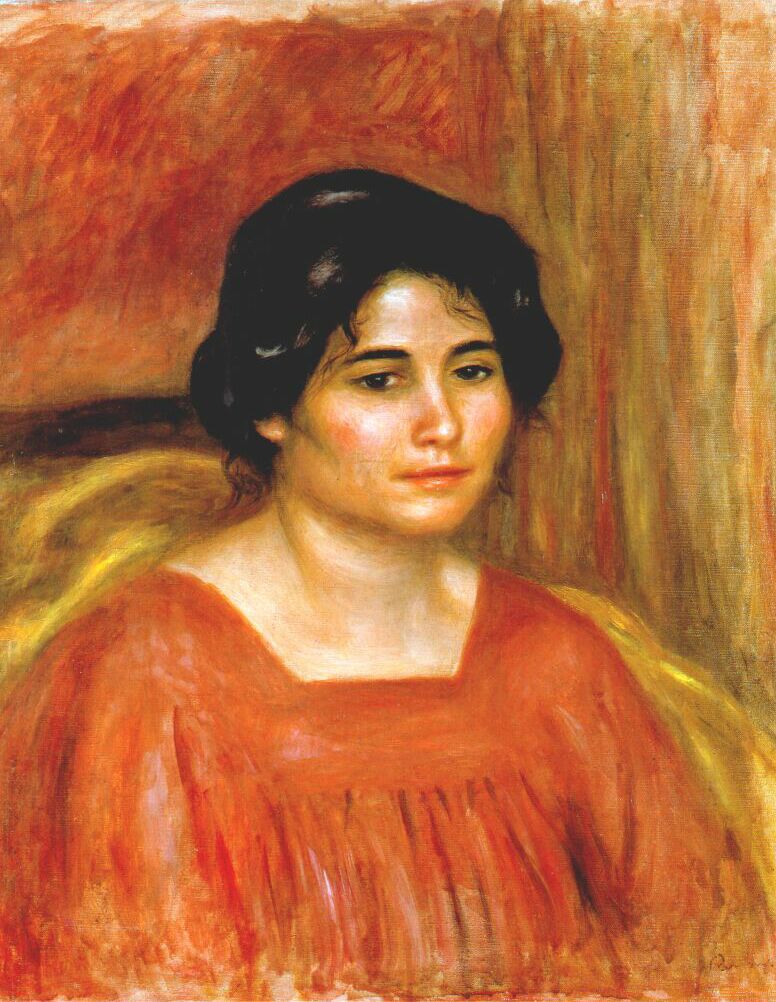This painting features a young woman, possibly in her late 20s or early 30s, seated in a golden chair. Her dark black hair is styled in an elegant updo, with a few tendrils softly pulled out. She wears a flowing orange dress that subtly harmonizes with the backdrop. The wall behind her is a gradient of warm hues, transitioning from a vivid orange on the left to a more muted yellowish-green on the right. Her expression is difficult to interpret, swinging between neutral and melancholic, with eyes that appear blank and emotionless, suggesting a sense of hopelessness or sadness. The woman is not looking directly at the viewer but slightly off to the side, adding to the sense of contemplative sorrow. The scene is devoid of any additional elements, keeping the focus entirely on her solemn presence, giving the impression that it might be a historical portrait from the 18th or 19th century.